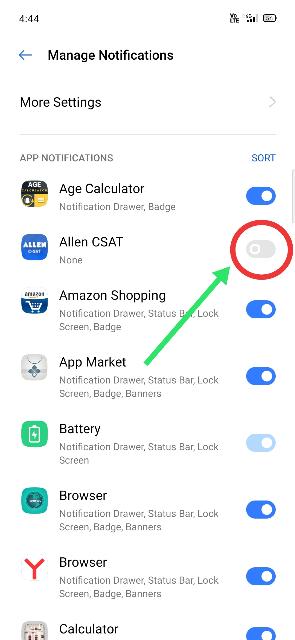The image is a screenshot of a smartphone's notifications settings screen. In the top-left corner, it displays the time as "4:44," while the top-right corner shows the standard battery and Wi-Fi icons. The background of the screen is completely white, with black font used for text. Directly beneath the time, the screen reads "Manage notifications," with a back arrow pointing to the left, indicating a way to return to the previous screen.

Below this, there is an option labeled "More settings." The main section of the screenshot is focused on the "App notifications" settings. Here, various applications are listed in gray text, such as "Age Calculator," "Alien Seasat," "Amazon Shopping," "At Market," "Battery," "Browser," and "Calculator." Each app has a toggle switch to the right, which users can use to enable or disable notifications. If the toggle is on, it appears in an aqua blue color; if off, it is grayed out.

Currently, all the toggles are blue (on) except for "Alien Seasat" and "Battery," which are gray (off). The toggle for "Alien Seasat" is circled in red, with a green arrow pointing towards it, likely indicating that this is a step-by-step guide on how to turn on notifications for the "Alien Seasat" app.

Overall, the screenshot exemplifies a typical notification settings screen on a smartphone, visually guiding users on how to enable notifications for a specific application.